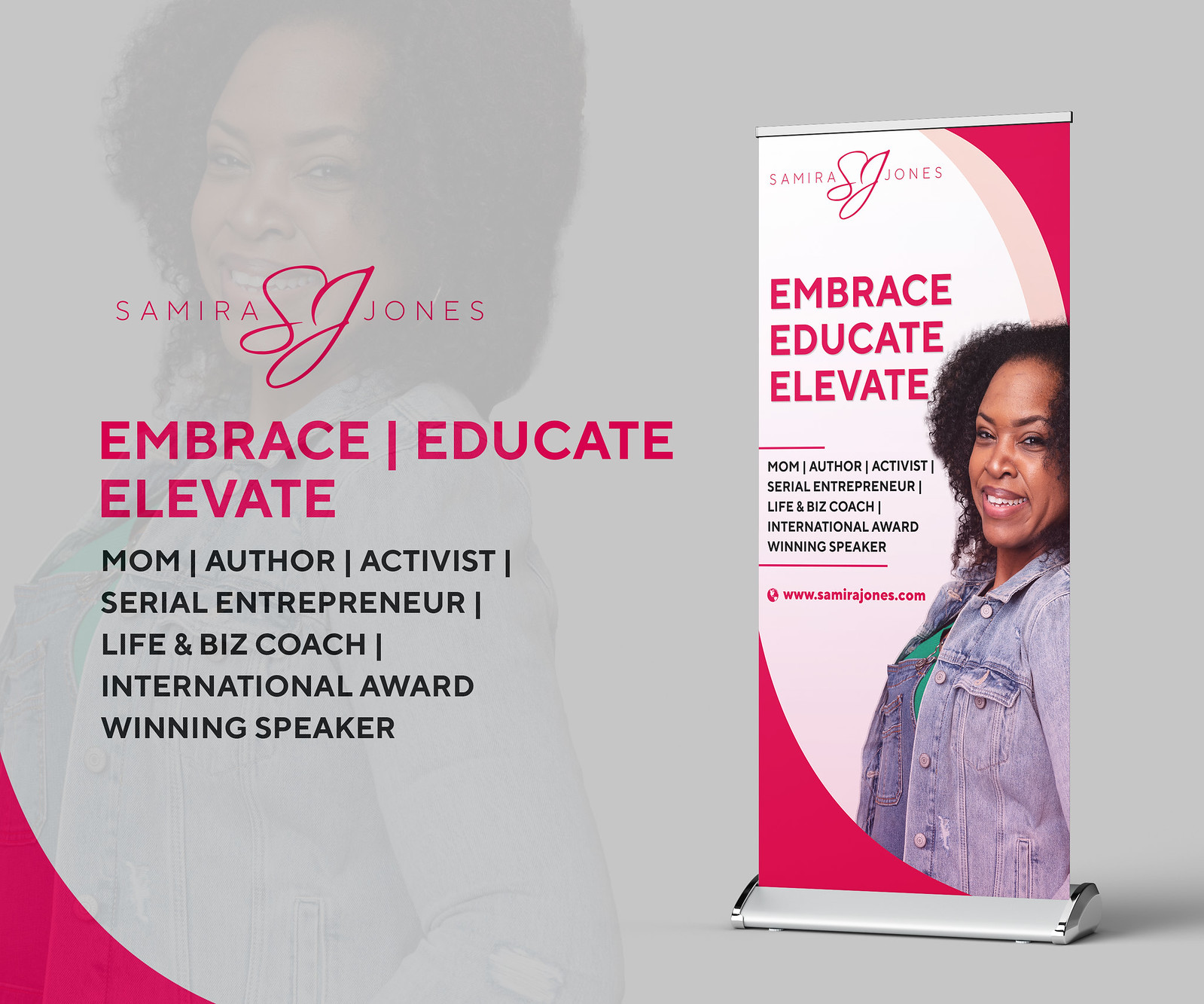This is a digitally created horizontal advertisement featuring motivational speaker Samira Jones. The image is divided into two halves, with a large vertical banner on the right displaying a prominent photo of Samira Jones against a gray background with a red corner on the bottom left. Her initials, "SJ," appear in cursive beside her name at the top of the banner, accompanied by the motivational slogan, "Embrace, Educate, Elevate," in bold red letters. Below this, in black text, are her various titles: "Mom, Author, Activist, Serial Entrepreneur, Life and Biz Coach, International Award-Winning Speaker." The left half of the image also contains her transparent photograph blended into the background, with repeating text listing her accolades, creating a cohesive and visually engaging promotional display.